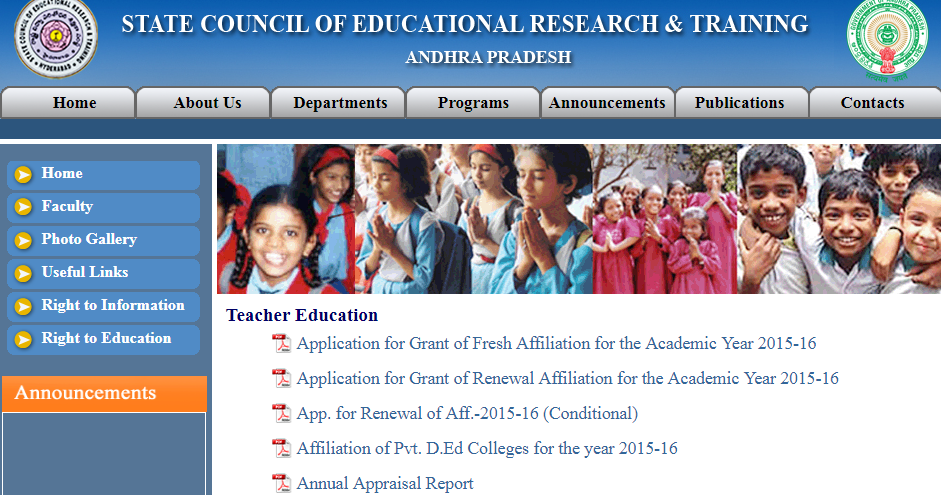The screenshot is taken from the website of the State Council of Educational Research and Training (SCERT), Andhra Pradesh. At the top left of the page, there is a distinctive logo featuring multiple concentric circles with various colors: a gray outer circle, a light purple inner circle, a red circle closer to the center, and a yellow dot at the very core. On the top right, there is another emblem consisting of a white outer circle, a dark green inner circle, a beige circle, and a central symbol resembling a turtle.

The website features a comprehensive navigation menu. At the top, from left to right, the tabs are: Home, About Us, Departments, Programs, Announcements, Publications, and Contacts. Additionally, on the far left sidebar, the options include Home, Faculty, Photo Gallery, Useful Links, Right to Information, and Right to Education.

In the bottom left section of the screenshot, there is an "Announcements" banner displayed in orange with white text. Meanwhile, at the top right, there is a vibrant image of a group of smiling children, adding a touch of warmth and positivity to the website’s overall design.